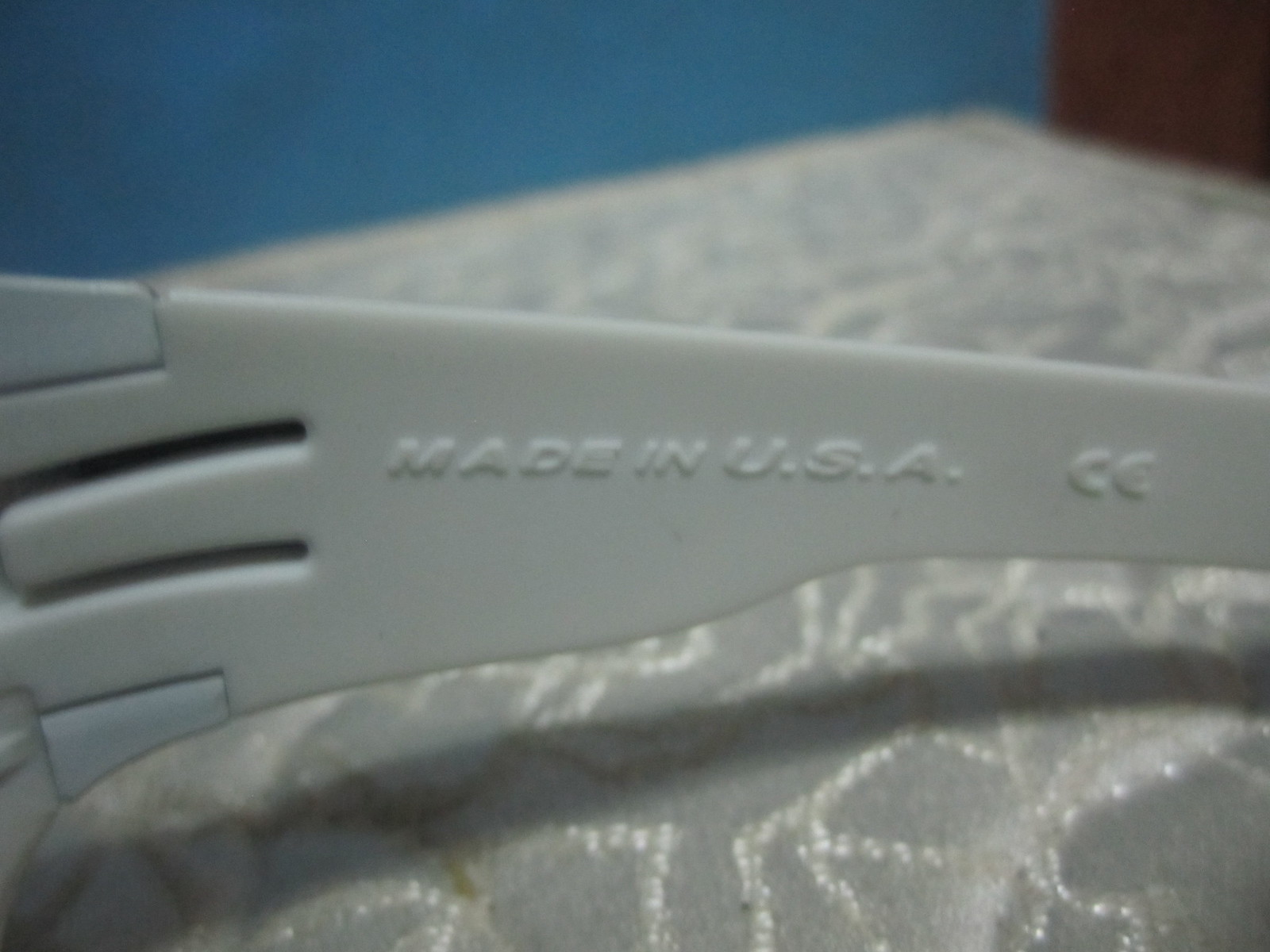The image depicts a close-up view of an unidentified object, focusing primarily on a section that appears to be part of the arm of a pair of glasses with distinctive characteristics. The glasses arm is primarily white, featuring gray joints at the front, which is wider, and tapering towards the back. Notably, the arm bears the inscription "MADE IN USA," followed by the characters "C" and "E." The object rests on a white, lace-like fabric, contributing to the background. The top portion of the image reveals a blue wall dominating the backdrop, with a smaller segment of brown, possibly a wooden cabinet or similar structure, seen at the top right. Despite some blurriness, the overall composition highlights the intricate patterns and design elements of the glasses against the pale, decorative background.